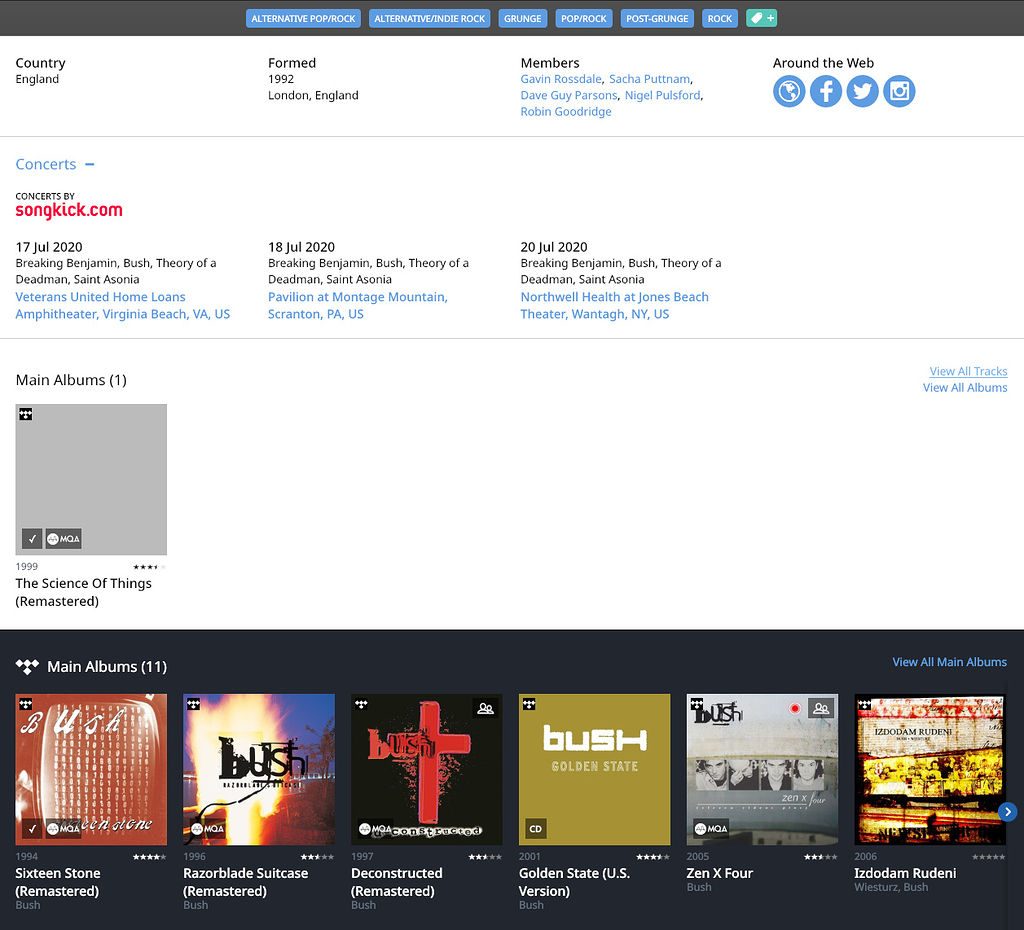### Detailed Caption:

This image is a screenshot of a music website, presenting a well-organized layout with distinct sections and color coding for better navigation. 

#### Header:
At the very top, a medium gray header spans the width of the page. Centrally aligned within the header are several tags, each enclosed in light blue rectangles with slightly rounded corners and white text. From left to right, these tags read:
- **Alternative Pop/Rock**
- **Alternative/Indie Rock**
- **Grunge Pop/Rock**
- **Post-Grunge**
- **Rock**

To the right of these tags, there is a teal rectangle with slightly rounded corners containing a white tag icon and a plus icon, indicating an option to add more tags.

#### Main Section:
The main section of the website has a clean white background and is divided into three segments by thin light gray lines.

1. **Information Section:**
   - **Header:** "Country, England, Formed, 1992, London, England, Members"
   - **Members List:** Each member's name is written in blue text: Gavin Rossdale, Satya Putnam, Dave Guy Parsons, Nigel Pulsford, Robin Goodridge.
   - **Around the Web:** Located to the right of the members list, this section features four icons with a light blue background, each representing different social media or web platforms. They include a white globe, a white 'F' (for Facebook), a white bird (for Twitter), and a white camera (likely for Instagram).

2. **Concerts Section:**
   - **Header:** "Concerts" written in light blue text, accompanied by a minus sign on the right for collapsing the section.
   - **Subheader:** "Concerts by" displayed in gray text, followed by "songkick.com" in red text.
   - **Concert Listings:**
     - **Event:** "17 July, 2020, Breaking Benjamin Bush Theory of a Dead Man, St. Esonia"
     - **Location:** "Veterans United Home Loans Amphitheater, Virginia Beach, Virginia, US" with the location written in blue text.

This detailed caption highlights the organized structure and the distinct sections of the music website, providing a comprehensive overview of its contents and layout.